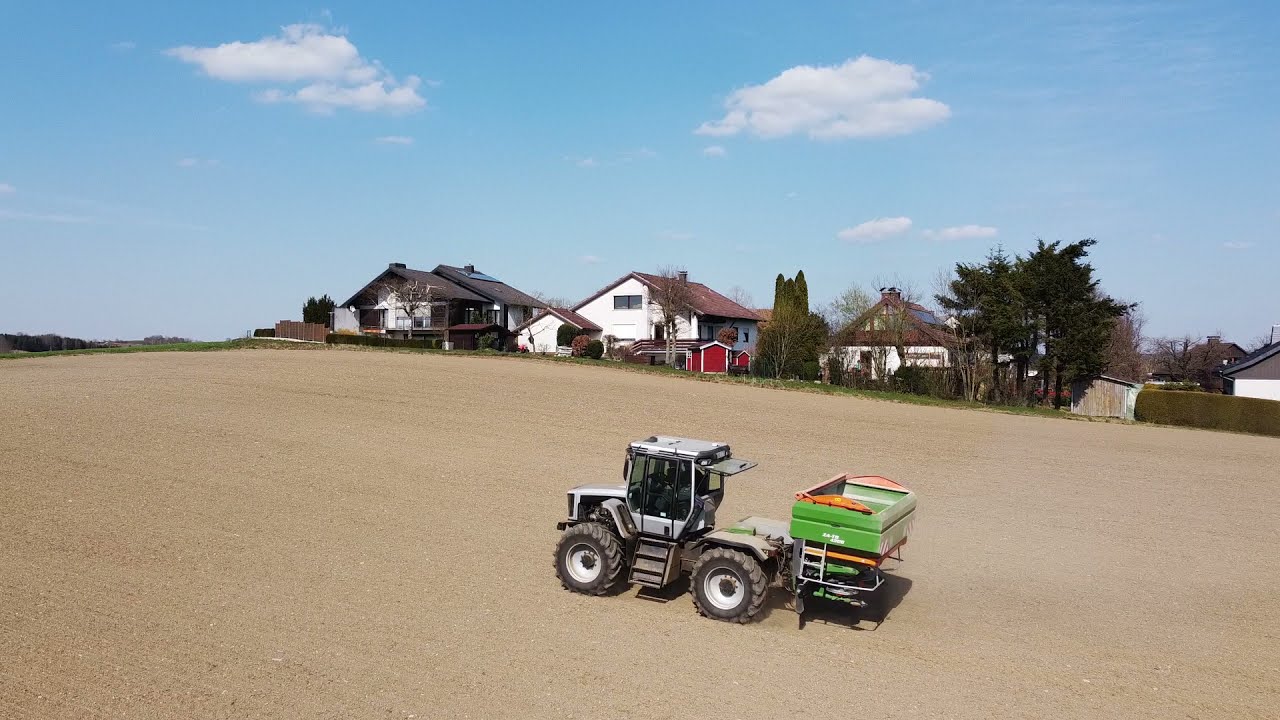The image depicts a vibrant rural scene featuring a recently plowed, light brown farmland on a slight incline, highest on the left and sloping down towards the right. At the center of the field, a white tractor with black wheels is driving, pulling a large green rectangular container. The tractor, characterized by its gray body and open-back cabin window, is well-lit under the clear, bright daylight.

In the background, a picturesque row of houses lines the horizon, each with distinct features. The houses primarily have white exteriors and terracotta or dark roofs that peak in a V-shape. To the left, there's a house with a darker facade and a black roof, contrasting against the predominantly white houses. Surrounding the houses are patches of greenery, including trees and bushes, with a hedgerow visible along the right-hand side of the field.

Above this serene countryside scene, the sky is a light blue adorned with a few wispy white clouds, adding a tranquil touch to the well-illuminated landscape.